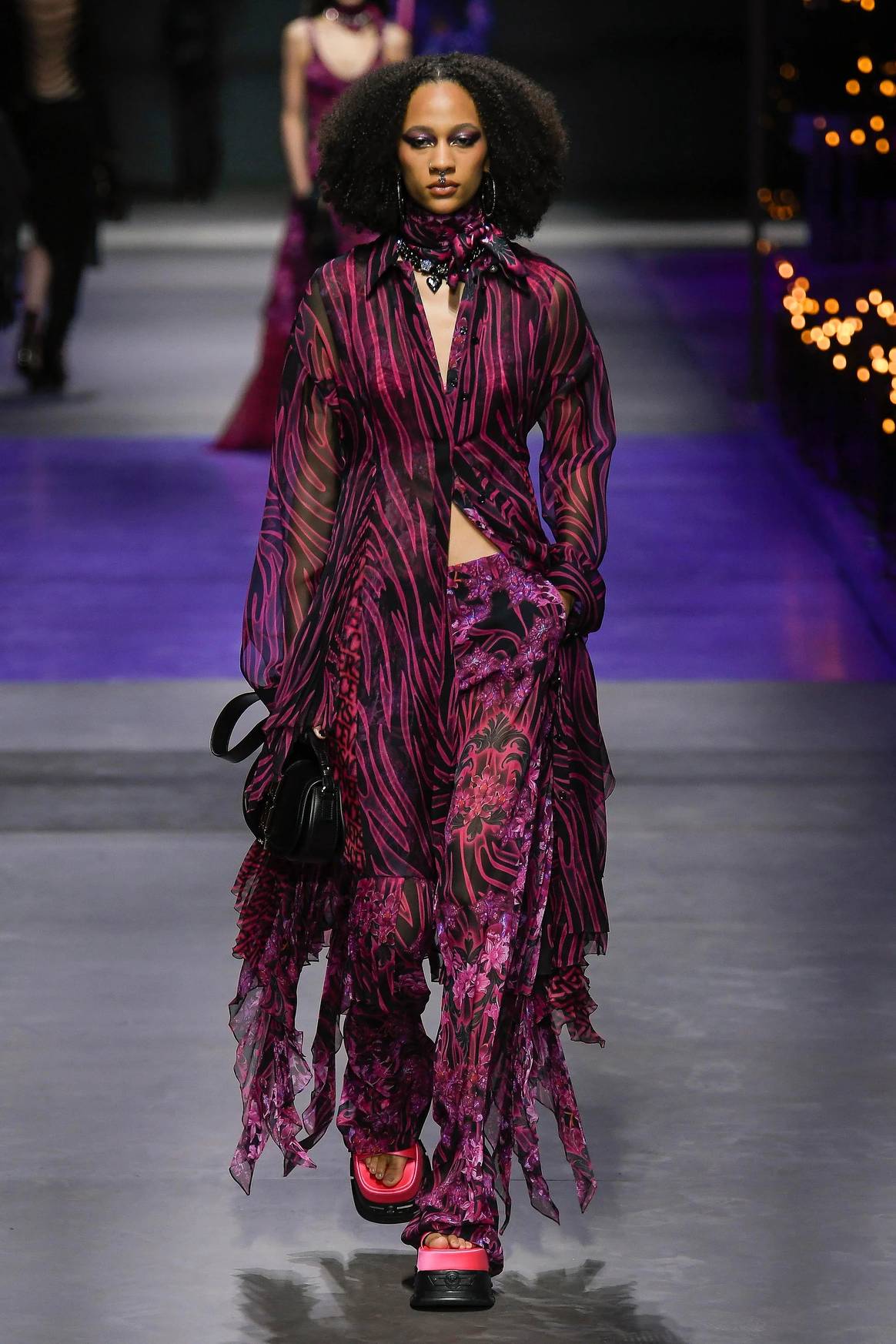This photograph captures a moment on a fashion runway, where a striking young black woman with shoulder-length, black, curly hair is the focal point. She exudes elegance in a long, flowing ensemble that combines deep magenta and black in a silky, sheer fabric. The ensemble features a long-sleeve button-down cardigan that opens just above her navel, revealing part of her midriff, and matching trousers that exhibit a magenta and black color palette. Her footwear consists of open-toed shoes with a stylish pink band accentuating the black base. She accessorizes with a chunky necklace and carries a sleek, shiny black handbag.

The runway itself is primarily gray, transitioning into a purplish hue and then back to gray at the rear. Adding to the ambiance are tiny, blurred lights in the background and distinctive orange lights on the right-hand side. In the background, another model is poised to take her turn, dressed in a maroon sleeveless dress. The scene is rich with the vibrant, dynamic energy of a high-fashion event, underscored by the dramatic play of colors and lighting.